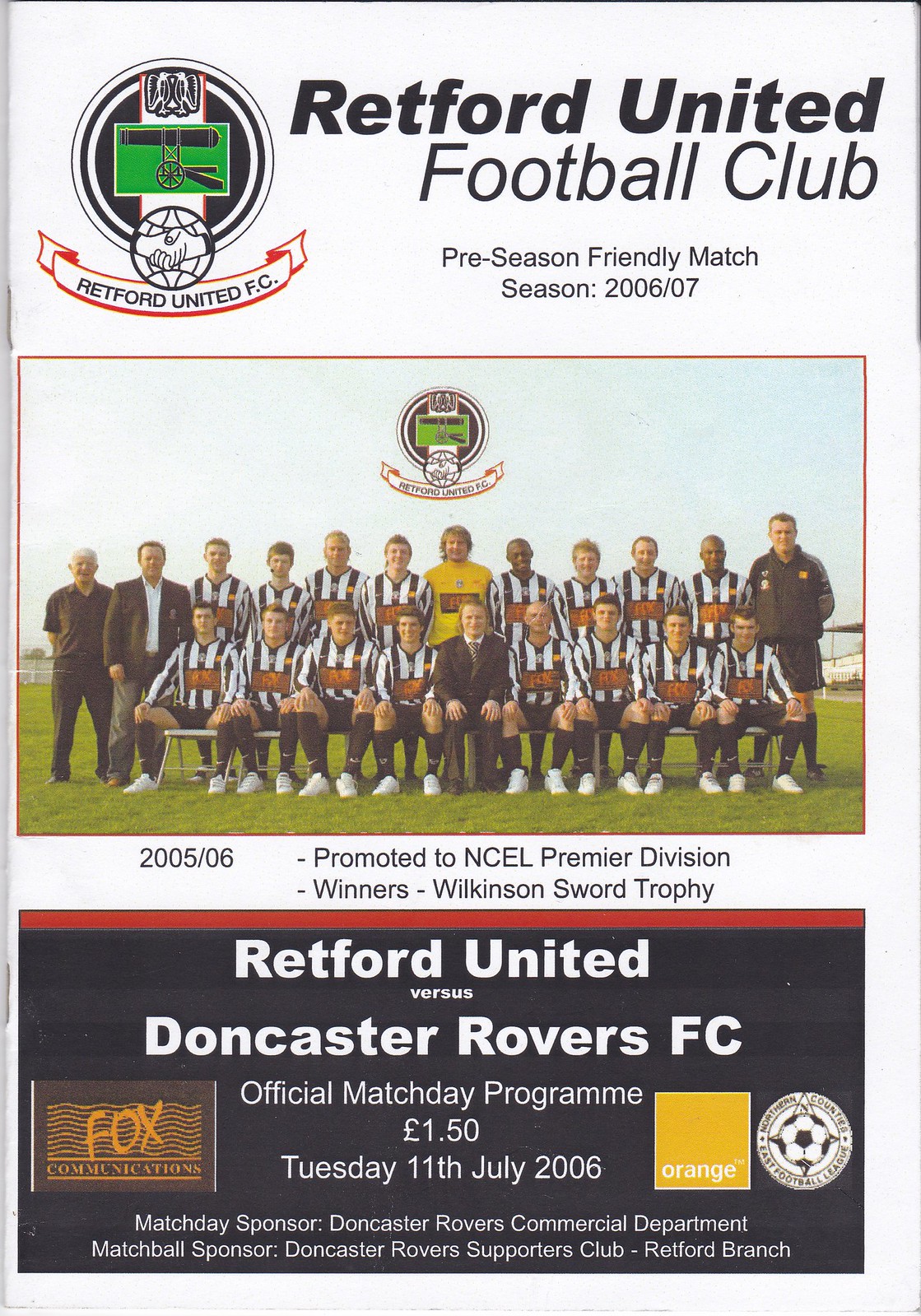The image depicts the cover of a promotional flyer for an upcoming football match. At the top, prominently displayed, it reads "Redford United Football Club Preseason Friendly Match Season 2006-07," accompanied by the Redford United FC crest. Below this headline, a photograph captures the full team, with players in black, orange, and white uniforms standing at the back, and more team members seated in front, centered around an individual in a suit, likely the team owner. The text beneath the photo celebrates Redford United's achievements, noting "2005-06 Promoted to NCEL Premier Division. Winners, Wilkinson Sword Trophy." Towards the bottom, on a blue background with a red stripe, essential match details are provided: "Redford United vs. Doncaster Rovers FC Official Match Day Program, 150 lbs, Tuesday, 11 July 2006," along with mentions of sponsors for the match day and ball.